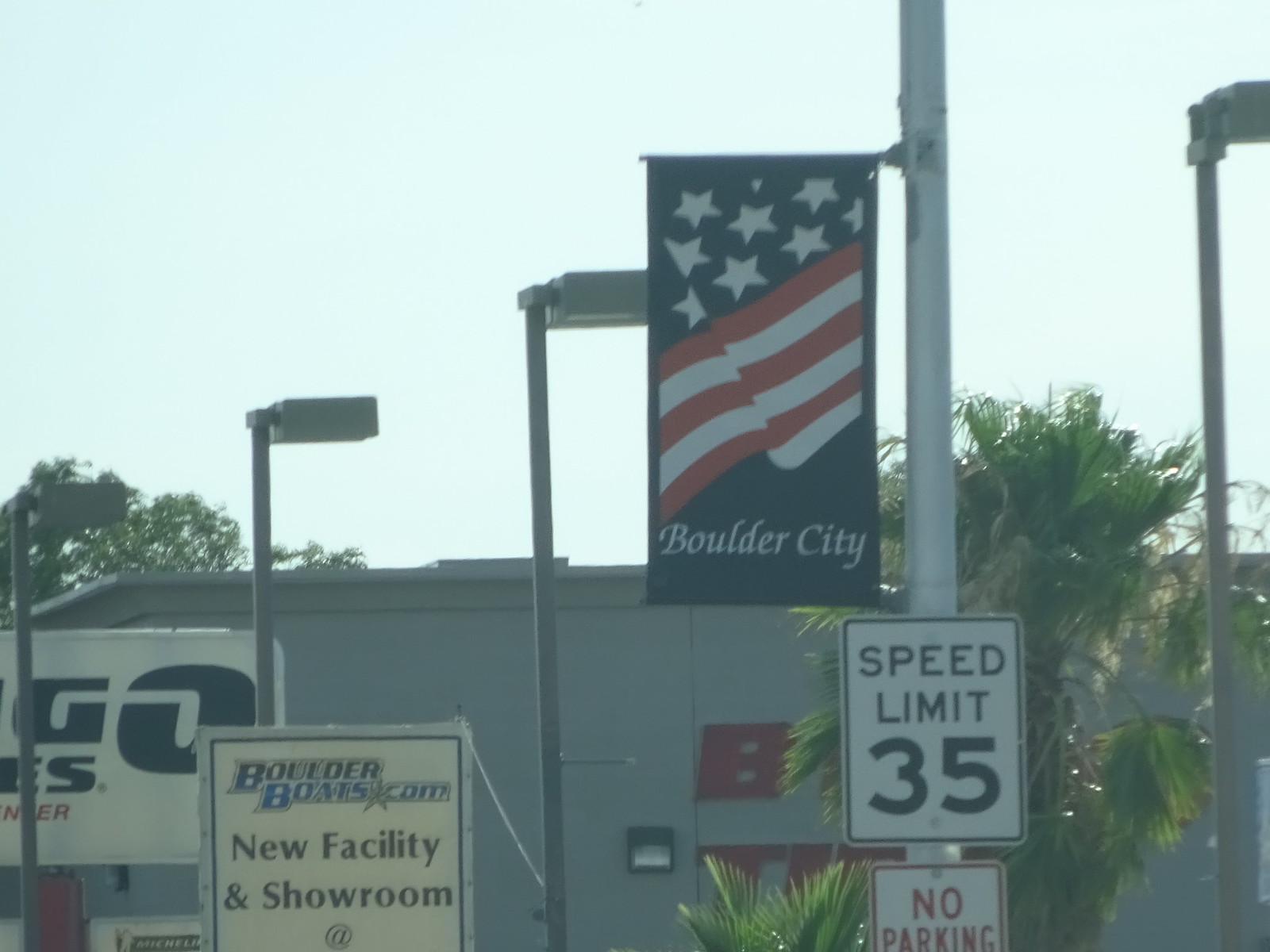In this rectangular, somewhat grainy and vintage-looking photograph reminiscent of the early 1980s, we see an exterior view of a gray building. The building features a partially obscured red sign, its text hidden behind several palm-like trees. At the forefront, there is a prominent white sign that reads "boulderboats.com new facility and showroom." To the right of the building, a silver pole stands with a rectangular white sign displaying a speed limit of 35. Below this, a second white sign with a red border reads "no parking." The sky above the gray building is clear, and green trees are visible in the background to the left.